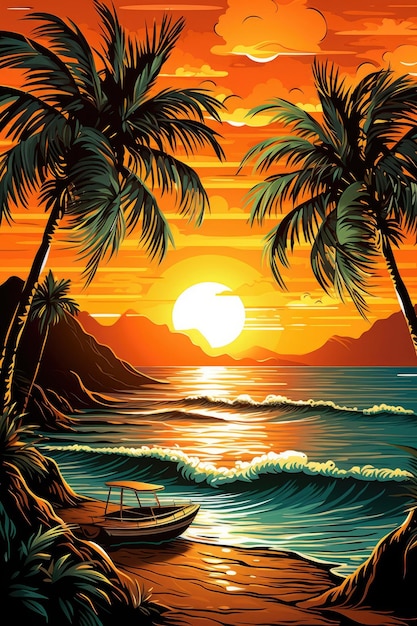This image is a detailed and picturesque digital illustration of a tropical beach scene at sunset, rendered in a clean, vector style with smooth lines. The vibrant sky, awash in gradients of oranges, reds, and yellows, is punctuated by fluffy, horizontal clouds and the radiant, white sun that sits just above the horizon. Framing the background are dark, reddish-orange mountains that outline the sun, creating a captivating halo effect.

In the midground, two towering palm trees with brown trunks and forest green fronds stand on either side, enhancing the symmetry and framing the sunset. The reflection of the sun's warm hues shimmers across the wet beach sand and the gentle waves of the turquoise ocean, which features white-capped waves rolling toward the shore.

The foreground is rich with detail, including patches of green vegetation and small brown hills on each side. A simple white boat with a yellow-orange roof, devoid of sails or a motor but equipped with handrails and four supporting poles, rests on the brownish sand. The boat’s nose points toward the right, subtly guiding the viewer’s gaze across the scene.

The meticulously crafted elements and the vibrant use of color make this illustration a stunning representation of a tranquil, tropical beach at sunset.